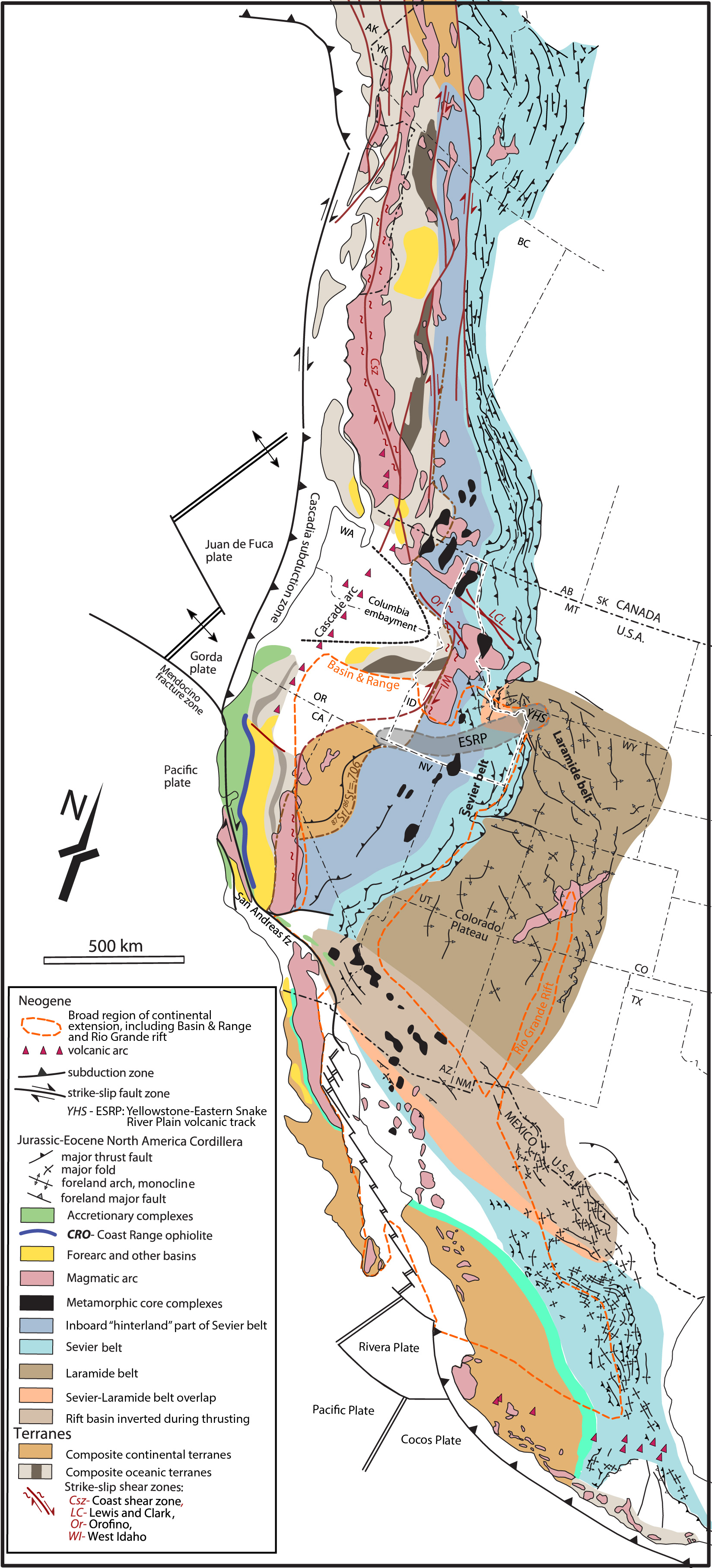The image depicts a detailed geological map of the western side of North America, spanning northern Mexico, the United States, and into Canada. Vibrantly colored, the map highlights various geological features, such as volcanic arcs, subduction zones, and fault zones. An extensive key located at the bottom left explains the colors and symbols, with red triangles indicating volcanic arcs and green regions representing accretionary complexes. Major geological features like the Colorado Plateau and the Rocky Mountains are prominently labeled. Specific color-coded regions include the pink magmatic arc, light blue Sevier Belt, brown Laramie Belt, and various shades of blue for different parts of the Sevier Belt. The scale bar indicates a distance of 500 kilometers, providing context for the map's scope. Dotted lines outline significant areas such as California, Oregon, Colorado, and British Columbia, underscoring the map's geological focus.